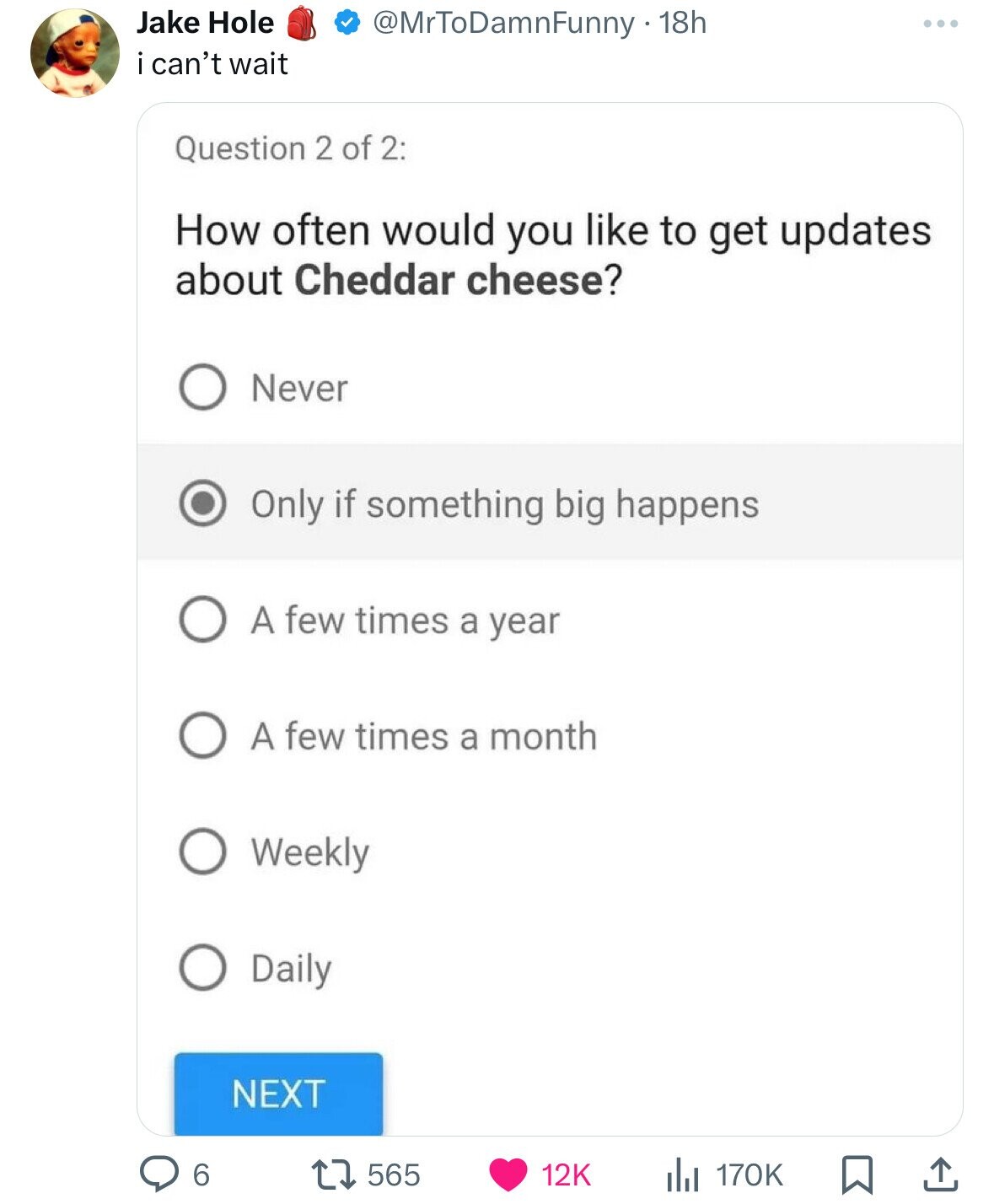Here’s the revised and detailed caption for the image:

"In this image, someone is filling out a questionnaire on their phone. At the top of the screen, there's a small profile picture visible, depicting what seems to be either a tiny person or possibly a cartoonish figure or even a very premature baby. The profile name displayed is either 'Jake Holt' or 'Jake Hole.' Adjacent to the profile, there is a red backpack icon and a verified checkmark. The username '@Mr.too.damn.funny' is listed along with a timestamp indicating the post was made 18 hours ago. Below that, in informal text, it reads, 'i can't wait,' with the first letter 'i' in lowercase. 

The main content shows 'Question 2 of 2' prominently in gray. Underneath, in black text, the question reads, 'How often would you like to get updates about cheddar cheese?' The available options for responses are listed with circular selection buttons next to them. The first option, outlined with a gray circle, says 'Never.' The next option, chosen by the user as indicated by a filled gray circle, reads 'Only if something big happens.' This is followed by other options: 'A few times a year,' 'A few times a month,' 'Weekly,' and 'Daily.' At the bottom right, there’s a blue 'Next' button for proceeding to the subsequent screen."